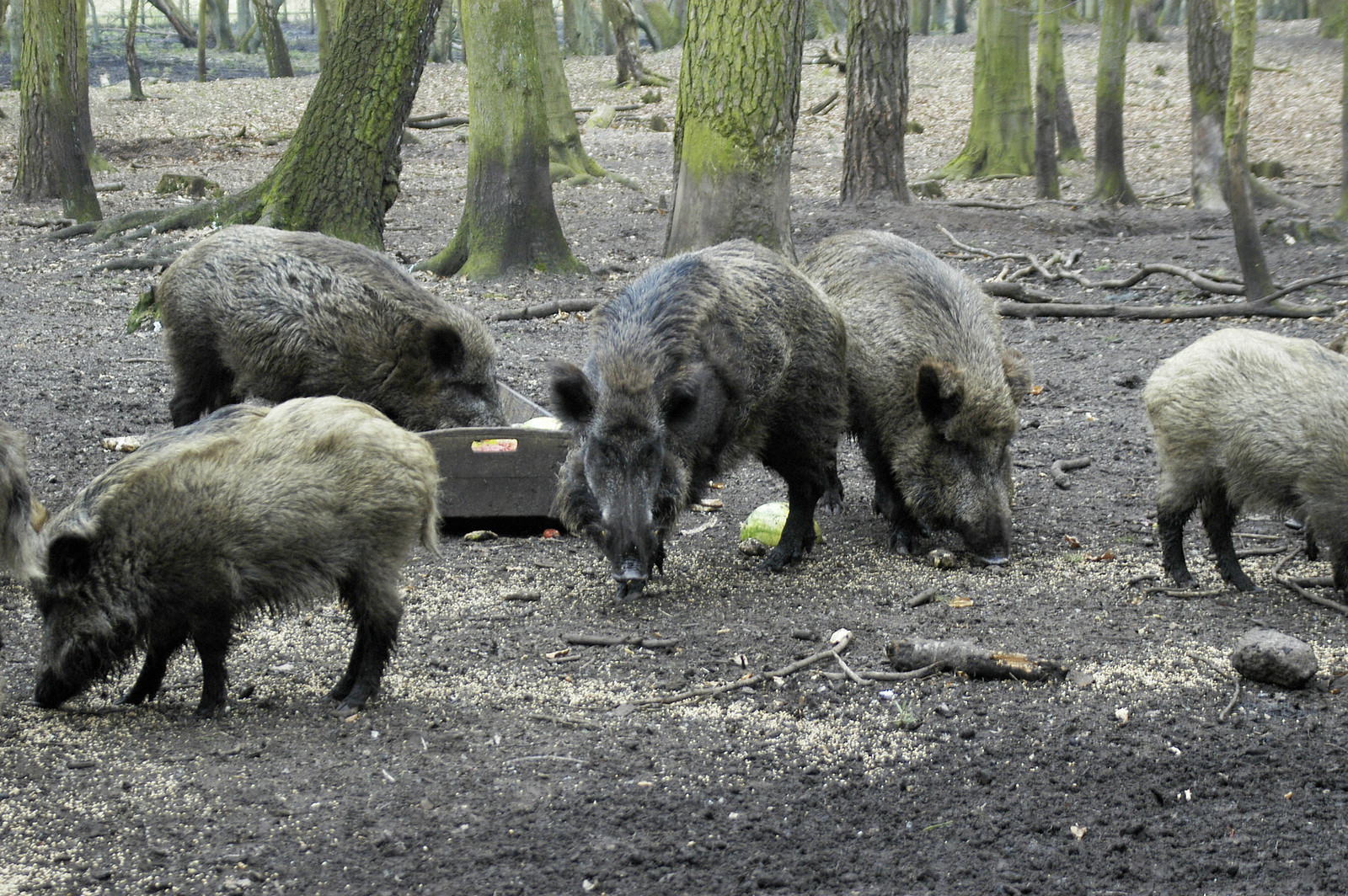The photograph captures half a dozen warthogs, reminiscent of Pumbaa from The Lion King, gathered around a rustic wooden trough brimming with food scraps, including colorful fruits and vegetables possibly watermelon or cabbage. The scene is set in a wooded area with numerous trees, characterized by grayish-brown trunks adorned with green moss and scattered twigs on the black, compacted dirt ground. The warthogs, varying in size and shades from very light gray to almost black, all possess dark faces, black ears, and hooves. One noticeably large warthog stands at the center, eating from the ground while peering directly into the camera, its menacing, pointed snout adding a foreboding feel to the group. Meanwhile, the smallest warthog, likely a juvenile of light gray color, stands on the far left, contrasting with its darker, larger counterparts. The presence of the wooden trough with metal handles, a green circular vegetable on the ground, and the seed scatter, suggests the warthogs might be in a captive setting within the woods.